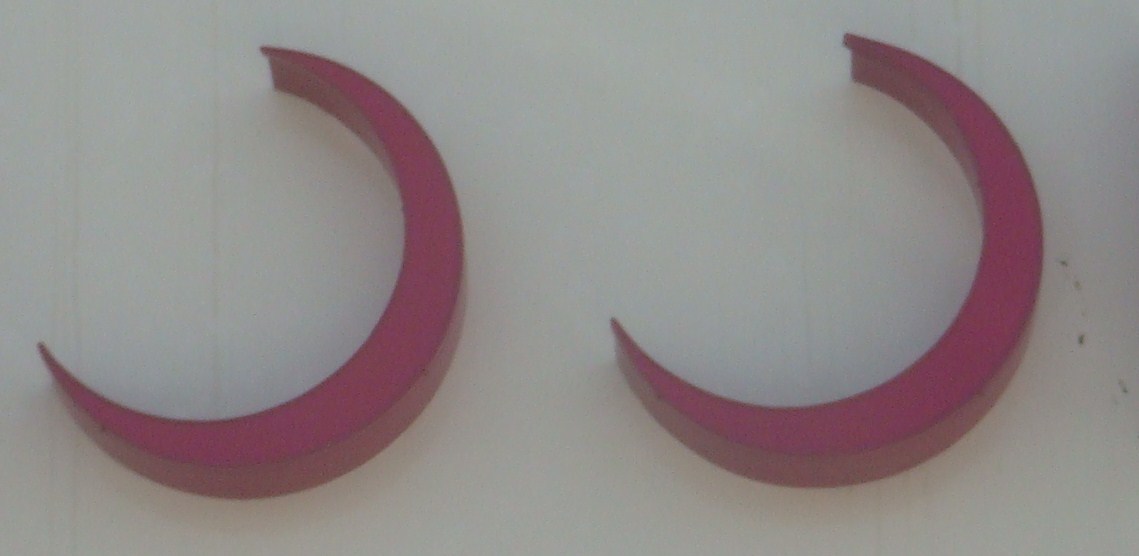This image features two identical, thick wooden crescent moon shapes, arranged side by side against a white backdrop. Each piece is stained in a mahogany red-brown, with a smooth, varnished finish. The crescents are positioned horizontally, oriented towards the upper left corner of the image. Measuring about two to three inches at their widest points, these shapes slightly resemble more than half circles or cut frisbees. With their consistent size and color, they stand out distinctly against the minimalistic background, creating a striking visual of geometric simplicity.